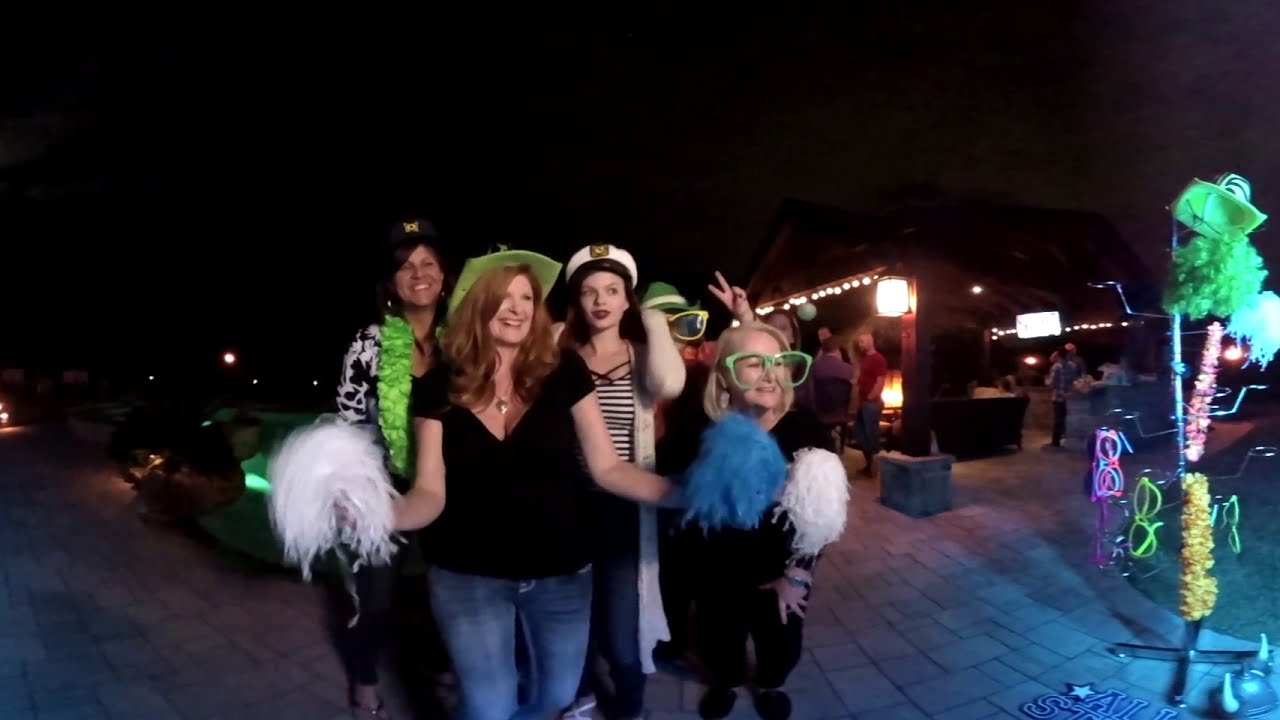The photo, taken outside at night, captures a lively group of five women posing together at a themed party. The women are dressed in festive attire, with several wearing green accessories hinting at a possible St. Patrick's Day theme, though one also wears a sailor's hat. Some women are holding white and blue wigs or pom-poms, and a few don oversized costume glasses.

In the background, the sky is almost entirely black, save for some gray clouds on the right. A well-lit pavilion with string lights and hanging lamps shelters several party attendees relaxing on patio benches. This backdrop includes a TV and a fire pit, around which people are gathered and chatting. To the left, there’s a seating area that appears to be illuminated with bright green light from below.

The foreground presents more playful details, including a stand adorned with green boas, assorted hats, and large, funny glasses, contributing to the party's whimsical ambiance. The ground beneath them is paved with square and rectangular stone tiles, adding to the outdoor setting's charm.